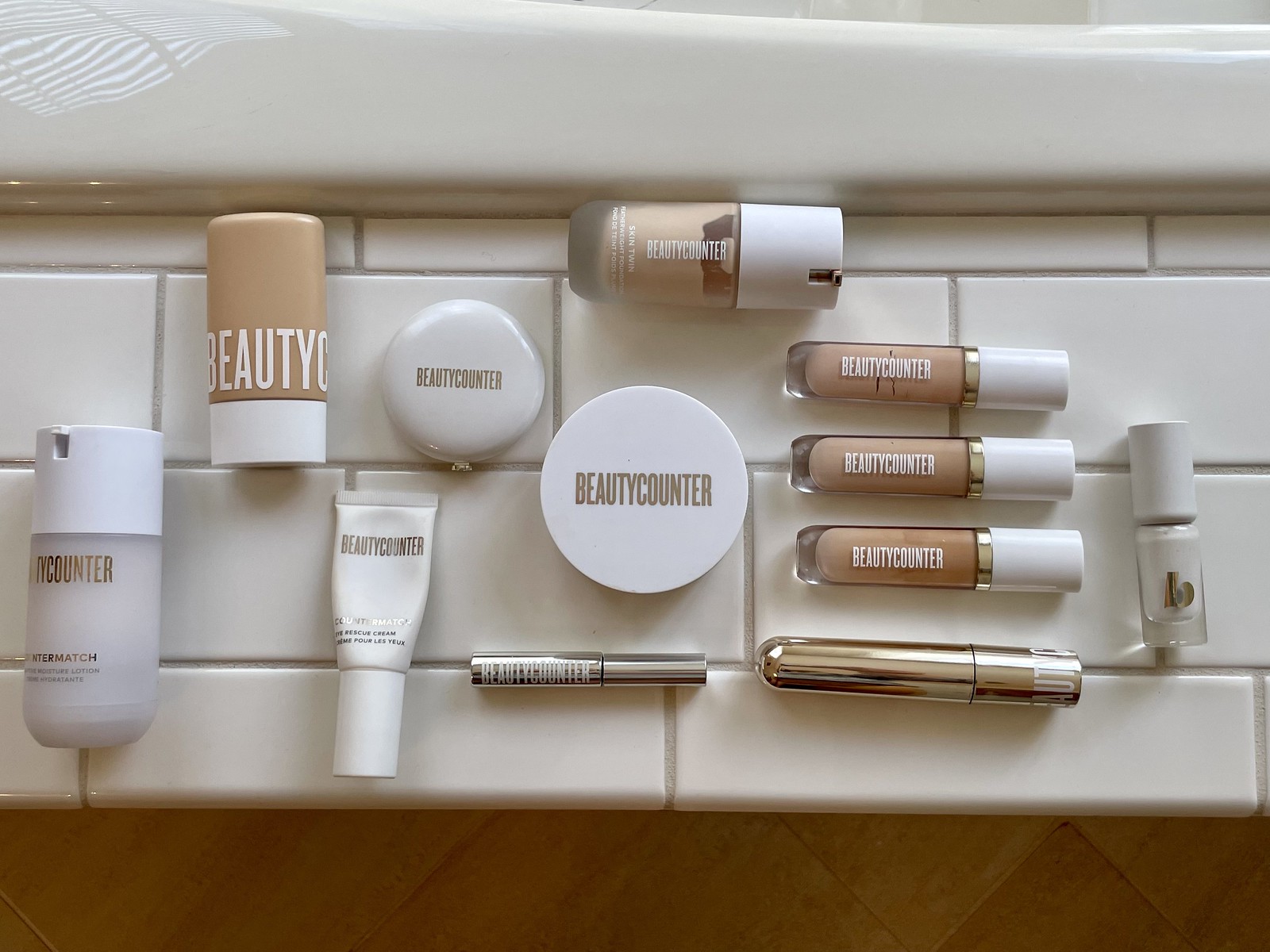In this image, a selection of beauty products is organized on a ledge, viewed from above. The ledge consists of a white base adorned with gray rectangular lines, framed by a brown floor at the bottom and a gray ledge at the top.

Starting from the left:
- A cylindrical container with the word "COUNTER" written in brown and capped with white.
- Next, a small tube labeled "Beauty Counter" in brown text.
- To the right, a flat, circular container also labelled "Beauty Counter" in brown.
- Below this, a tube of lip gloss.
- Following are four narrow, rectangular containers: the bottom one is bronze-colored while the top three are brown. All are marked "Beauty Counter" in white and have white caps.
- Further to the right is a very small container with a white cap.
- Above this, another flat, circular container.
- To its left, a brown container with a white cap.
- At the very top, another brown container with a white cap completes the layout.

This arrangement of beauty products offers a varied and neatly organized display, framed by a gray ledge at the top for background contrast.